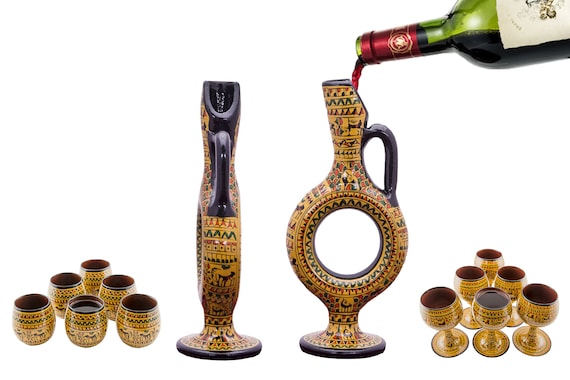The image depicts an arrangement of uniquely styled objects set against a completely white background. Central to the composition are two identical, tall, giraffe-shaped vessels that feature a mosaic-like pattern with vibrant colors, including yellow and red zigzags and dots. These vessels have handles and circular, hollow centers resembling a donut shape, and each rests on a flat base. In front of the vessel on the right, red wine is being poured from a green bottle.

Surrounding these giraffe-shaped vessels are various matching cups. On the far right and far left sides of the image are small stemless tumblers and goblets, all of which are decorated in a consistent Egyptian-inspired design that complements the central objects. The overall scene is well-lit with natural light, making the intricate details and vivid colors of the patterned surfaces clearly visible. The symmetrical arrangement and the cultural aesthetic of the items create a visually striking and organized composition.